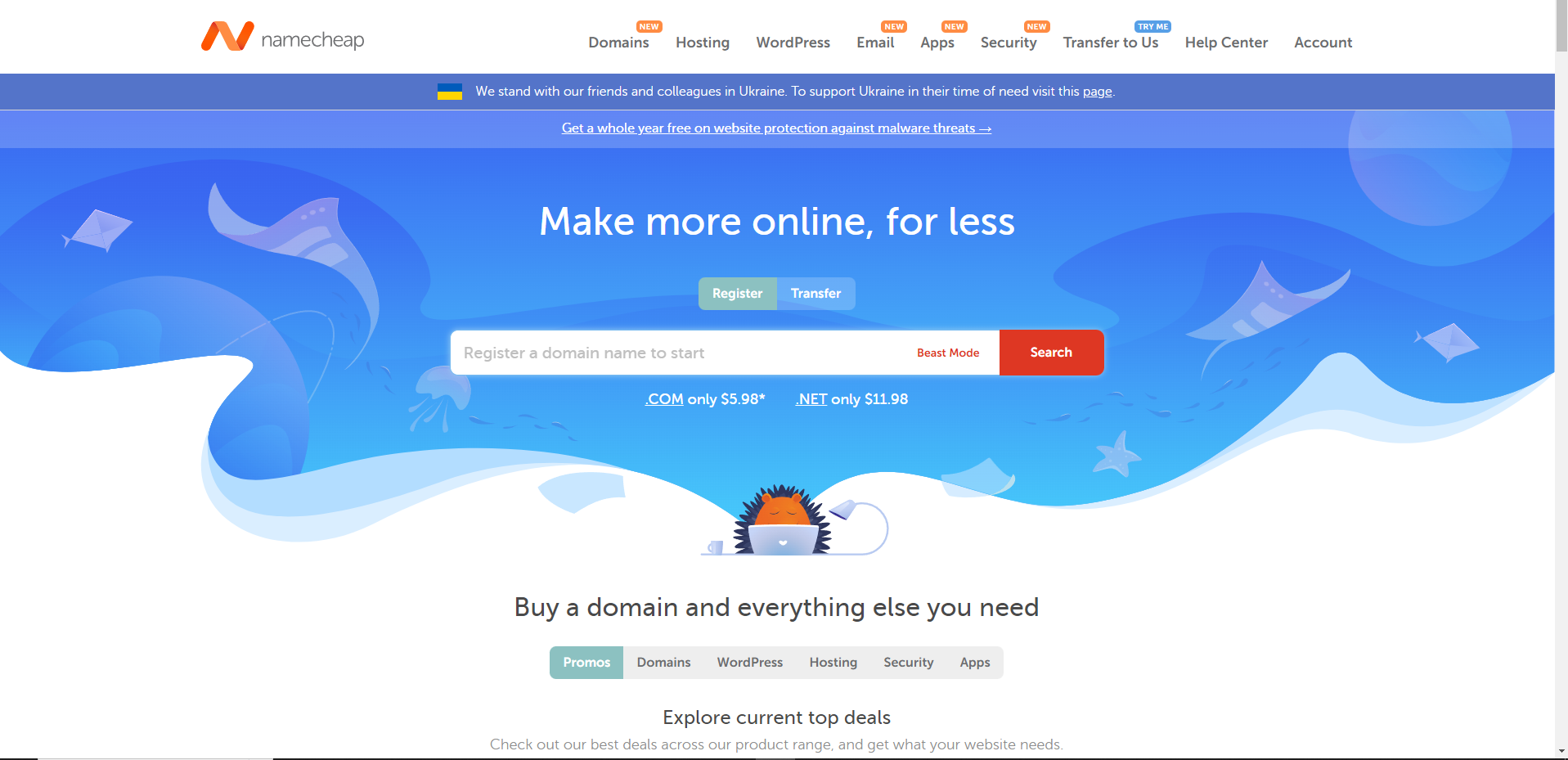This web page belongs to the company Namecheap. In the top left corner, there's a capital 'N' composed of red and orange lines forming the letter 'N,' followed by the company name 'Namecheap' in thin, lowercase black text. Running horizontally across the top of the page are navigation options including 'Domains,' 'Hosting,' 'WordPress,' 'Email,' 'Apps,' 'Security,' 'Transfer to Us,' 'Help Center,' and 'Account', all set against a white background.

Below this, a thin, bright blue ribbon stretches across the page, featuring the Ukrainian flag and white text stating, "We stand with our friends and colleagues in Ukraine. To support Ukraine in their time of need, visit this page," with the word "page" in bold. Underneath, a lighter blue ribbon of the same width highlights an offer in white text: "Get a whole year free on website protection against malware threats," accompanied by a forward arrow.

Central to the page is a bold message in white text reading, "Make more online for less." Directly below this are two prominent buttons: a gray button labeled "Register" and a blue button labeled "Transfer." A white search bar follows, containing the prompt "Register a domain name to start." To the right within the search bar is a red button labeled "Search."

Beneath the search bar, in white text, .com domains are promoted at "only $5.98" and .net domains at "only $11.98." Adjacent to this information is an endearing graphic of a hedgehog (or possibly a porcupine) sitting at a silver laptop. Finally, the phrase "Buy a domain and everything else you need" is displayed in black text below the graphic.